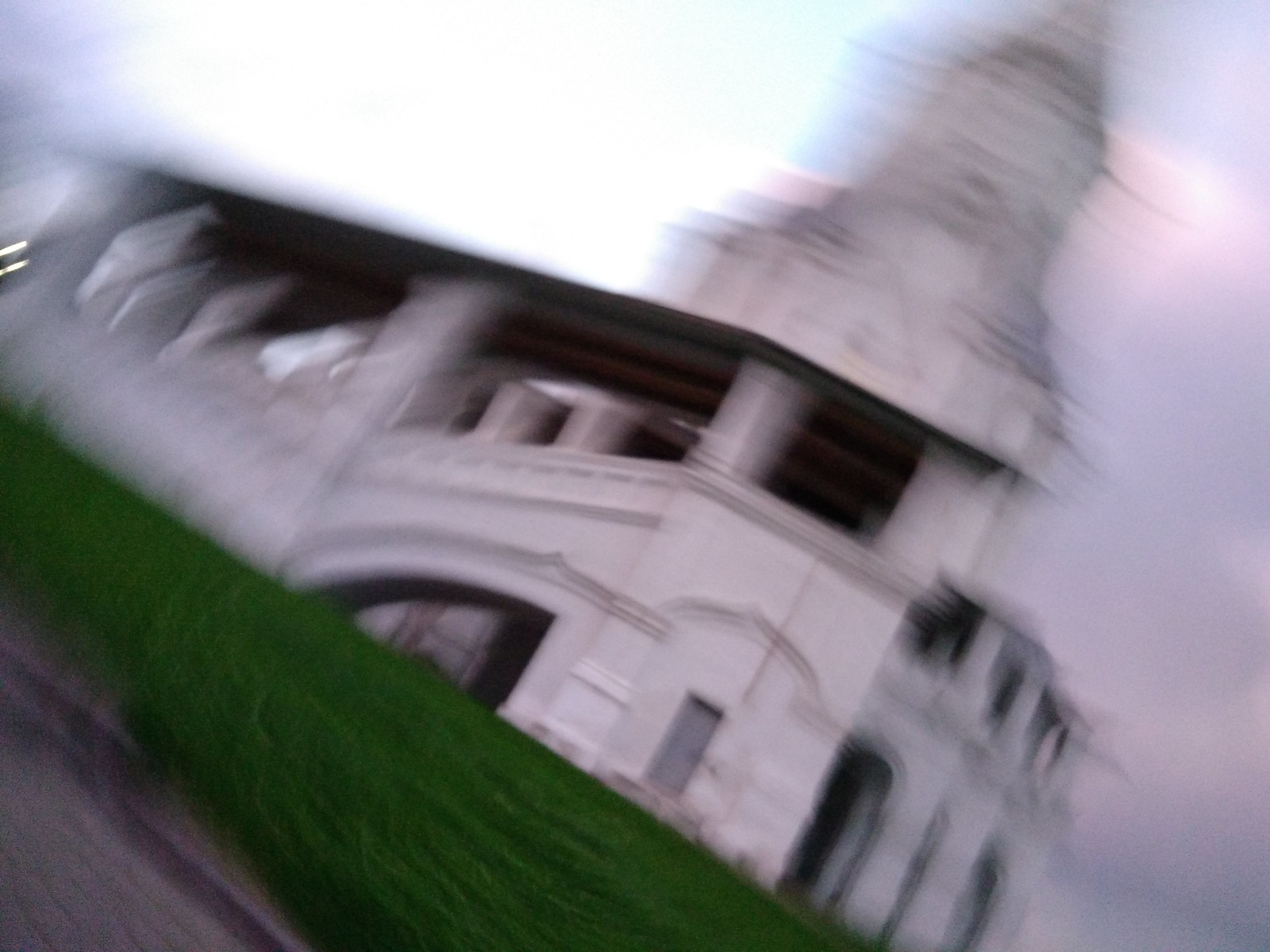A highly blurred photograph of a white building taken at a pronounced diagonal angle, with the upper left corner sloping towards the bottom right. The image is so out of focus that specific architectural details are indiscernible. However, the structure appears to feature a bell-shaped element at the top, possibly a decorative or functional architectural piece. The building’s façade is gray, likely a result of the blur, and includes a main entrance and several arch-shaped doorways with rounded tops. The left side of the building is particularly indecipherable due to the blur. Beneath the structure is a patch of green grass, adding a streak of color. The background includes a partially visible sky on the right side, while the left side is dominated by an overexposed white flash, obscuring any details in that area.